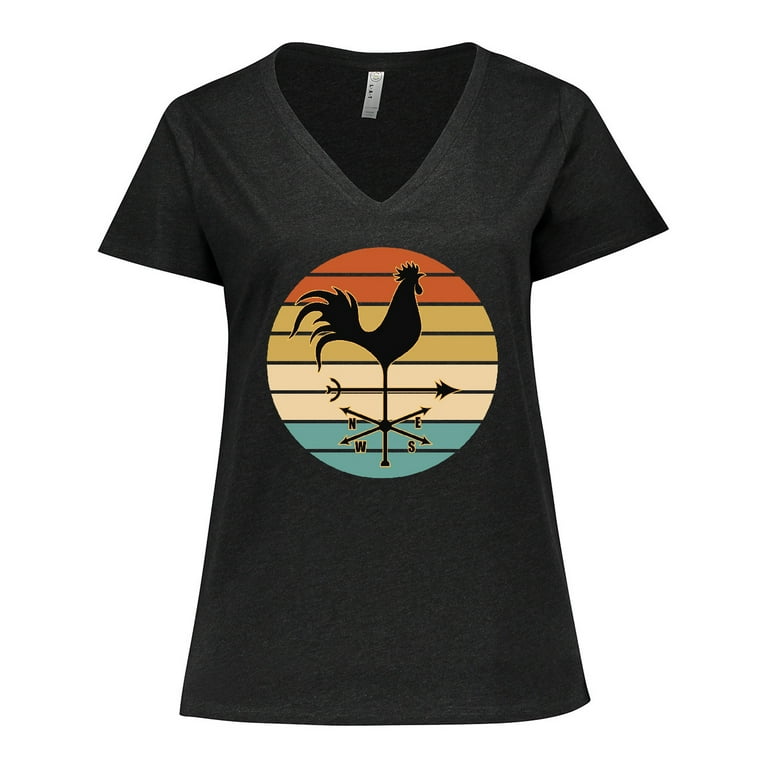This is a professionally taken, color photograph of a dark charcoal gray, almost black, short-sleeved, v-neck t-shirt, likely designed for women given its tapered middle. The t-shirt is set against a plain white background, emphasizing the garment. A white label is visible at the back of the neck. Centered on the shirt is a distinctive graphic within a circle, featuring horizontal stripes in a sequence of colors: brownish orange, light brownish yellow mustard, white, and light blue. A black silhouette of a rooster in profile is prominently displayed at the top of the circle, atop a weather vane that points right, marked with the letters NW, E, and S.